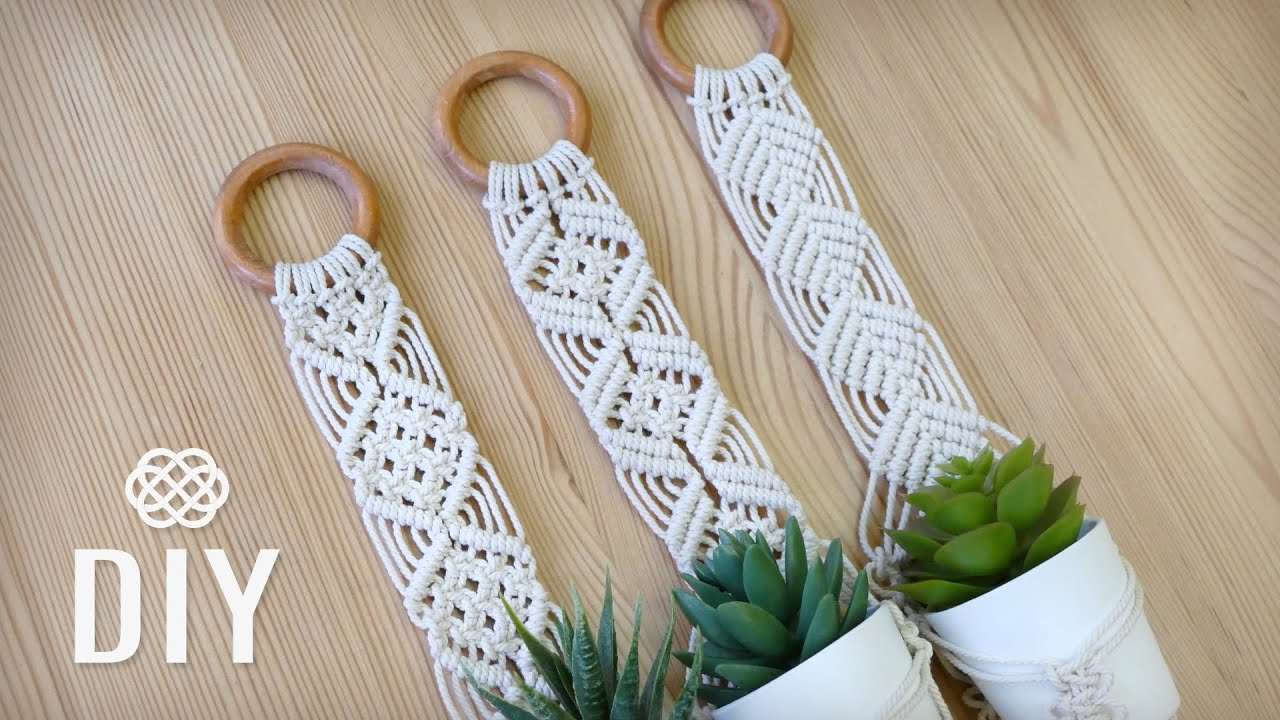This color photograph, likely from a blog, showcases a DIY project involving three macrame plant hangers laid on a pale whitewashed diagonal wooden floor. In the bottom left corner of the image, "DIY" is prominently displayed in bold white letters below a logo resembling a knotted or Celtic design. Each macrame hanger, intricately woven into triangular patterns with slight variations, features a wooden hoop at the top. The hangers collectively support small, featureless white pots, each containing a different variety of realistic-looking fake succulents. The consistent use of wooden rings and the elegant simplicity of the planters highlight the cohesive yet unique nature of this handmade project.